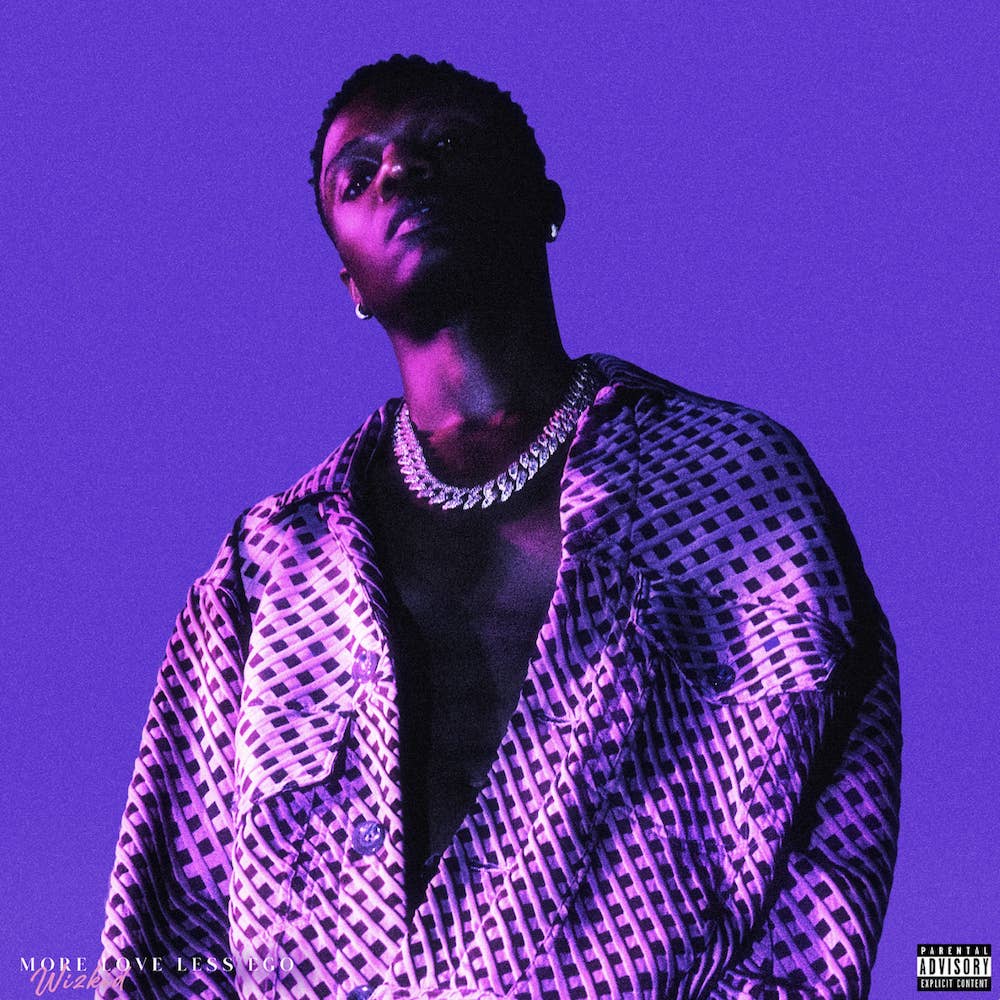The image appears to be the album cover for Wizkid's "More Love, Less Ego." The background is a vibrant lilac or purplish color, giving the image a striking and modern feel. In the center, an African American man, likely Wizkid, is posed confidently with his chin slightly raised and head gently tilted askew. He sports diamond hoop earrings in both ears and a prominent silver chain link necklace around his neck. The man's shirt, a geometric or basket weave patterned garment, is an oversized button-up that is open to expose much of his chest. This shirt also features buttoned front pockets and long sleeves. To add to the luxurious flair, the shirt seems to be crafted from a silky material. Text is situated on the lower part of the image: "More Love, Less Ego" in an all-caps, elevated font is on the bottom left in white, with "WIZKID" beneath it in a handwritten-style pink font. To the bottom right, there is a black and white Parental Advisory label indicating explicit content.